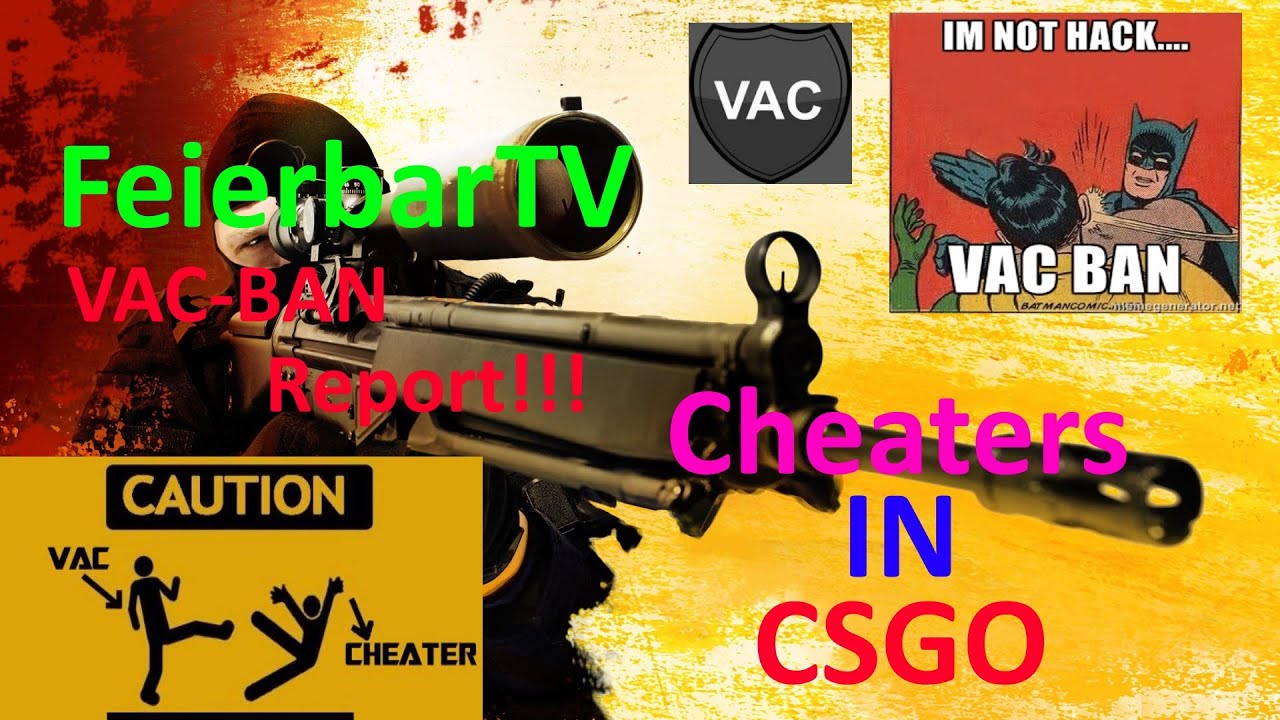The poster features a man dressed entirely in black, including a black hat and mask, prominently holding a long, black sniper rifle. The background is a gradient, with red on the left, transitioning to bright pale yellow in the middle, and yellow on the right. Noteworthy text appears on the man's face in three lines: the first line in green reading "Fire Bar TV," the second line in red stating "VAC haven't been banned," and the third line indicating "Report." In the top right corner, there is a red mini-poster depicting Batman slapping Robin, with the text "I'm not a hack" and "VAC ban on." In the bottom left, there's a mustard yellow rectangular section labeled "Caution," with an illustration of a stick figure labeled "VAC" kicking another labeled "Cheater." Additional elements include the words "Cheaters in CSGO" beside the gun barrel and a gray shield with "VAC" in white text next to the Batman image, referencing the anti-cheat system used in the game Counter-Strike: Global Offensive (CSGO).